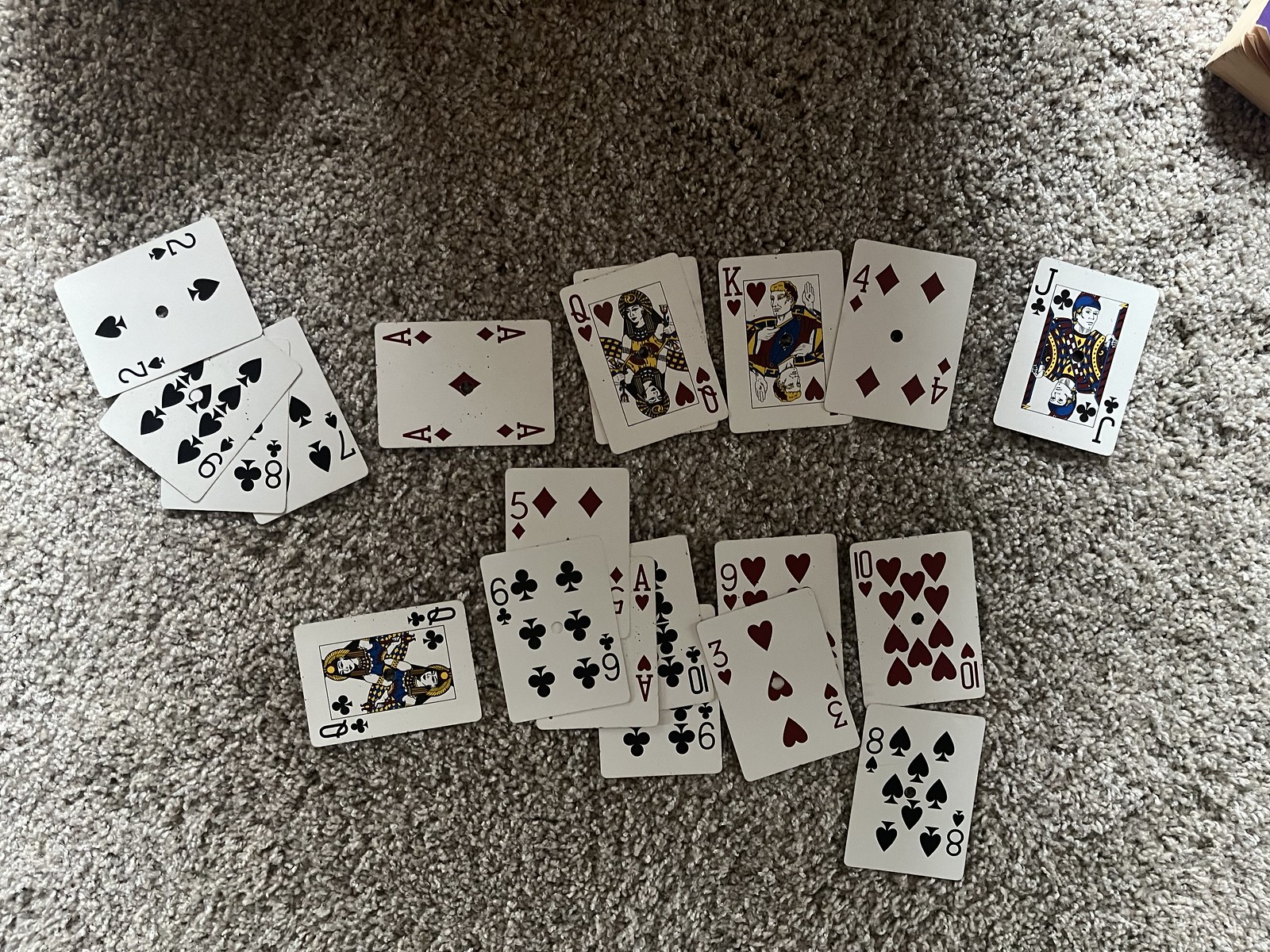An overhead view of a collection of playing cards arranged on a gray carpet, revealing intricate details under the shadow cast from above. In the top right corner, the edge of a small book with a blue cover and white pages peeks into the frame. The playing cards are spread out in two distinct rows. 

In the top row, starting from the left, there is a sequence of the Seven, Eight, Nine, and another Seven of Spades. To their right, lies an Ace of Diamonds placed sideways. Next, a six-faced die rests mid-frame, followed by the King of Hearts, Four of Diamonds, and the Jack of Clubs positioned at the far right.

The bottom row features a Queen of Clubs oriented with its top facing left. Adjacent to it is a slightly overlapping stack: the Six of Clubs with a Five of Diamonds partially visible underneath. Below and to the right of the five is an Ace of Clubs, and further right, a Ten of Clubs. Directly underneath the Ten is a Nine of Clubs. Continuing to the right, a Nine of Hearts sits adjacent, with a Three of Hearts slightly overlapping its bottom edge. Finally, the row concludes with a Ten of Hearts to the right and an Eight of Spades just below it.